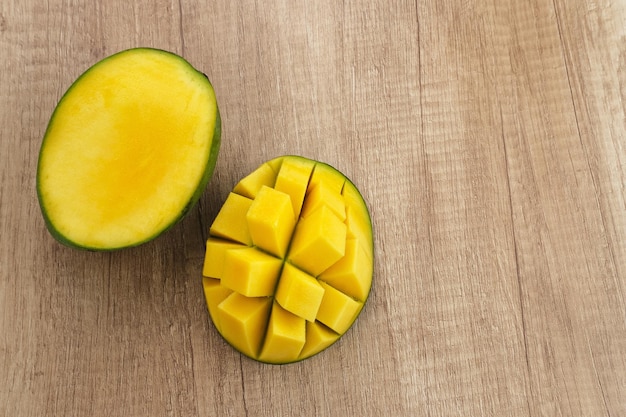In this indoor kitchen scene, a light wooden or distressed cutting board features prominently. Displayed on the board is a yellowish fruit, possibly a mango, though its exact identity is uncertain. The fruit has been cut in half, with the left half remaining largely intact and smooth inside. The right half has been intricately diced into small squares while still attached to the skin, suggesting it's prepped for easy consumption. The setup, bathed in soft indoor lighting, underscores the simple, everyday beauty of food preparation.